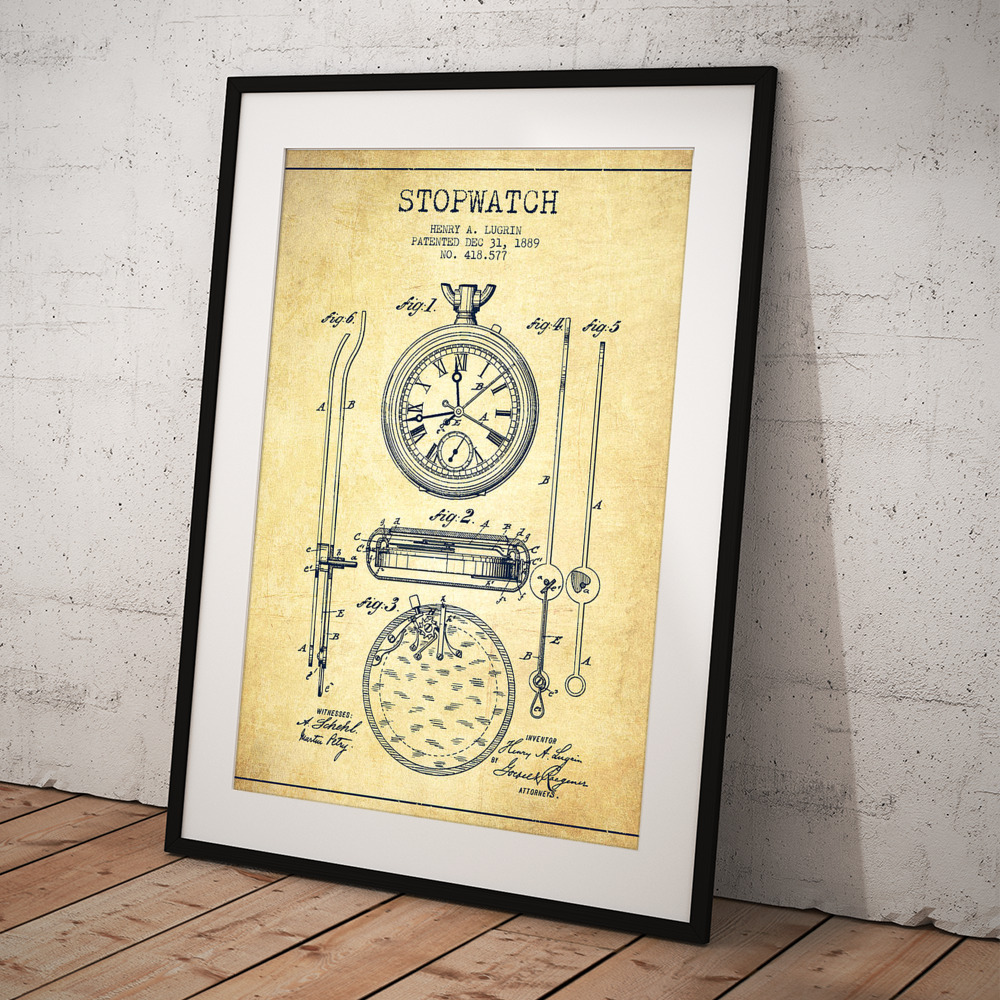The photograph captures a framed illustration of a detailed diagram, reminiscent of those found in vintage textbooks or patent documents. The diagram, set against a yellow background, meticulously displays the components of a stopwatch, with portions and figures distinctly labeled. Titled at the top, the illustration attributes the invention to Henry A. Lugren and notes the patent date as December 31, 1889, with patent number 418577. The figures illustrate various views and internal workings of the stopwatch, including its face, sides, and internal mechanisms, alongside signatures presumably from the patent office. The print is enclosed within a white mat and a black frame, leaning against a textured white stucco wall. The setup rests on a wooden floor with medium to light brown grains. The professional quality of the illustration suggests it might be an advertisement for this particular framed print, potentially featured in a magazine, catalog, or on a web page.